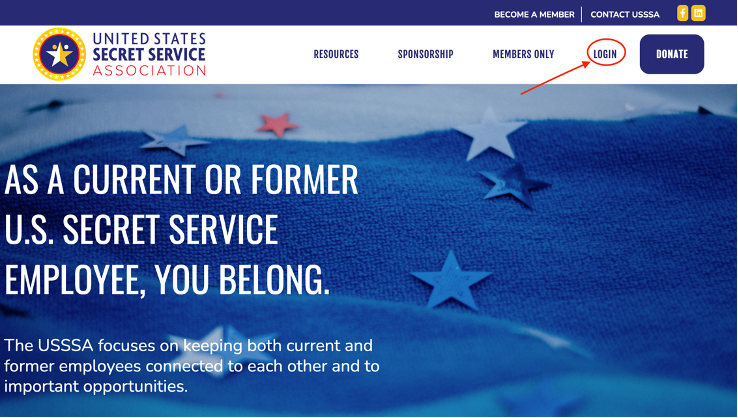In the upper left corner of the image, the text "United States Secret Service Association" is prominently displayed. Moving right, the navigation menu includes options such as "Resources," "Sponsorship," "Members Only," "Login," and "Donate." The "Donate" option stands out with white text on a blue rectangular button. The "Login" button features blue text on a white background, emphasized with a red circle and arrow pointing to it, suggesting a focus on educating users to log in at that location. The navigation bar itself is dark blue with a lighter blue strip at the top. On the right side of the navigation bar, additional options include "Become a Member" and "Contact USSSA," alongside yellow buttons for Facebook and LinkedIn.

Below the navigation bar, a photograph features prominently, showcasing striped blue and white fabric with metallic paper stars scattered across it. Positioned in the left center of the image, a bold statement reads, "As a Current or Former US Secret Service Employee, You Belong," in the largest font and all capitals. This emphasizes the inclusive nature of the organization. Below, in smaller white text, it states, "The USSSA focuses on keeping both current and former employees connected to each other and to important opportunities," highlighting the association's mission of fostering connections and providing opportunities.

The overall color scheme includes shades of blue, white, and accents of metallic and red. This image appears crafted for educational purposes, guiding users on how to log in and emphasizing the association's commitment to its members.